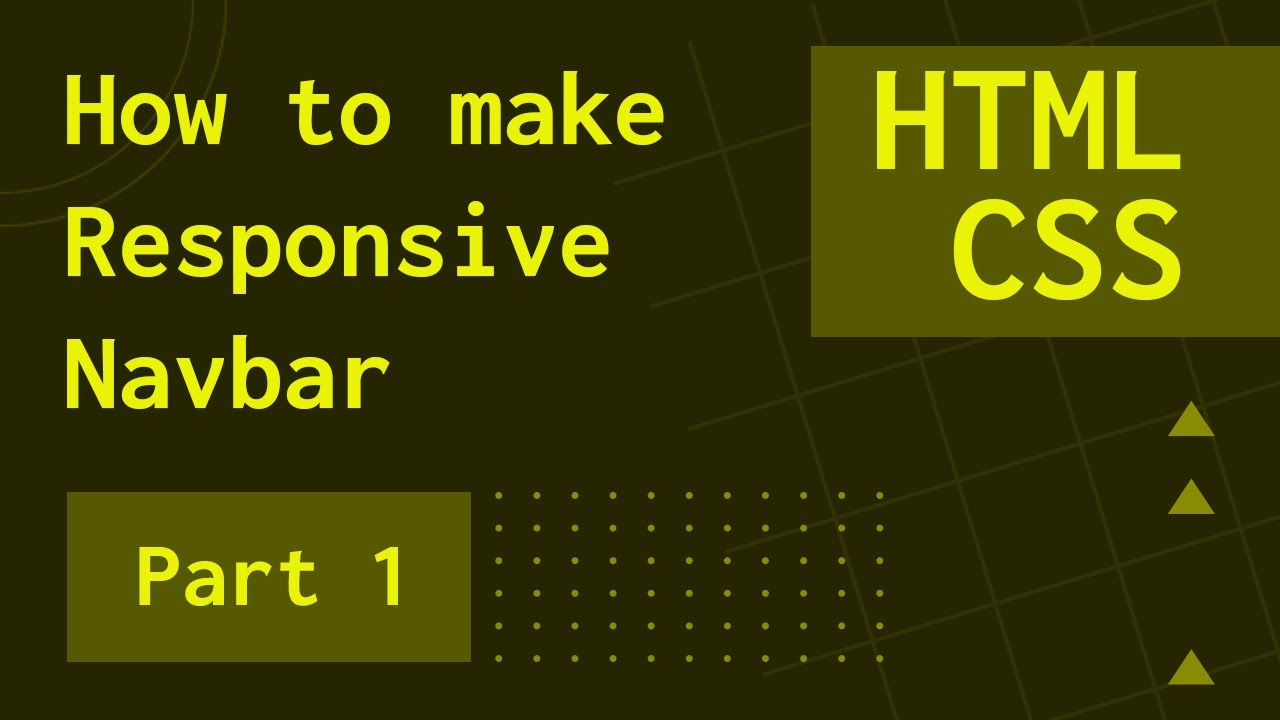Here is the cleaned-up and detailed descriptive caption for the image:

---

The image features a simple rectangular layout with a lime green font. Starting in the upper left-hand corner, the text reads "How to Make" in one line, followed by "Responsive" on the next line. Beneath "How to Make," the word "Responsive" is repeated. Below the second "Responsive," the text "Nap Bar" is written, all in the same font and lime green color.

Towards the center of the image is a dull green, grayish-brown rectangular block. To the right of this block, a grid of lines stretches in a 7 by 13 arrangement, seven lines running vertically and thirteen horizontally. Positioned atop this rectangular block is the text "Part One" in lime green.

The background of the entire image is a dark, muddled brownish-green. In the upper right-hand corner are two semicircles placed equidistant from each other. Starting in the lower right-hand corner and extending up to the upper middle section of the image is a crosshatch grid pattern.

Additionally, in the upper right-hand corner, there is another dull green, rectangular block. On this block, the text "HTML CSS" is written in all capital letters and in light green. In the lower right section of the image, there are two closely spaced triangles with their tips pointing upward, and a third triangle in the lower right corner that also points upward, with approximately an inch of space separating it from the two triangles above.

---

This should provide a clear and structured description of the image.